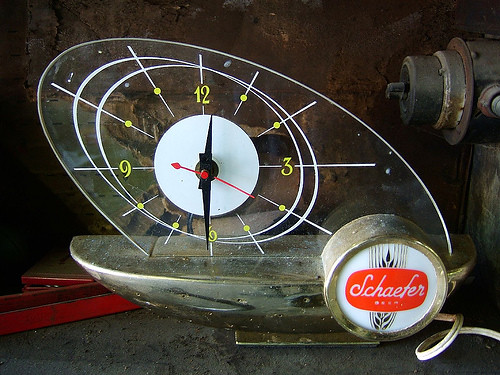The image features an elegant analog clock with a transparent, oval-shaped casing that extends from the bottom left to the top right. The clock face prominently displays the numbers 12, 3, 6, and 9 in gold, with gold dots representing the other hours. A white circle in the center houses the black hour and minute hands, alongside a red second hand. The clock is mounted on a rounded, brown wooden base. On the bottom right of the base, there is a small white circle with a red rectangle in the middle, emblazoned with the brand name "Schaefer" in white text. The clock's background reveals a deteriorating brown wall, and a white electrical cord is visible at the bottom right corner of the clock. Additionally, there is an antiquated mechanism resembling a drill emerging from the top right of the clock. To the left of the clock, a mysterious red object, possibly a metal pole, is partially visible.